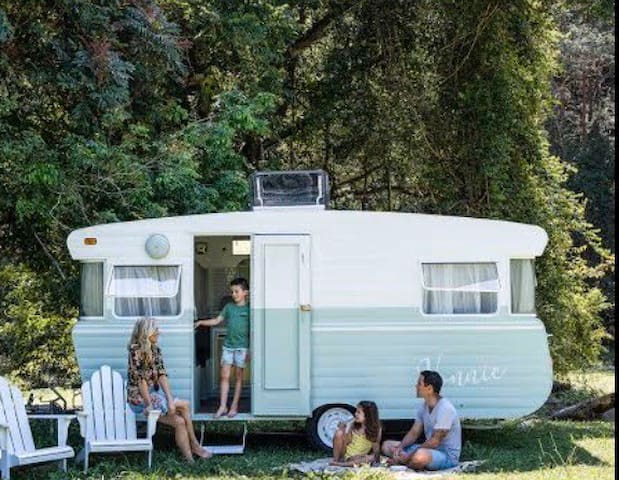In this detailed outdoor scene, a family of four is captured relaxing beside a vintage hitch camper from the 1950s or 1960s, painted in a two-tone scheme of white and very light green or pale blue. The small trailer, approximately 16 to 20 feet in length, has one set of wheels and features several open windows and an open doorway for ventilation. 

A blonde woman, sporting long hair, shorts, and a colorful shirt, is seated just outside the camper, gazing at her young son who stands in the doorway. The boy, dressed in blue shorts and a green shirt, faces his mother from the partially open door. Two white Adirondack chairs are positioned nearby, adding to the cozy ambiance.

On a blanket spread out on the grass, a man and his daughter are seated near the back wheel of the trailer. The man wears a white top and blue shorts while the little girl is dressed in yellow. This relaxed family scene unfolds against the backdrop of a natural wooded area filled with green foliage.

The camper has lettering on its side—possibly the word "Venice" or a sequence of characters resembling "V, W, I, C"—though the exact text is obscured. This idyllic moment captures a peaceful escape in the woods, with the family enjoying the simple pleasures of outdoor life.